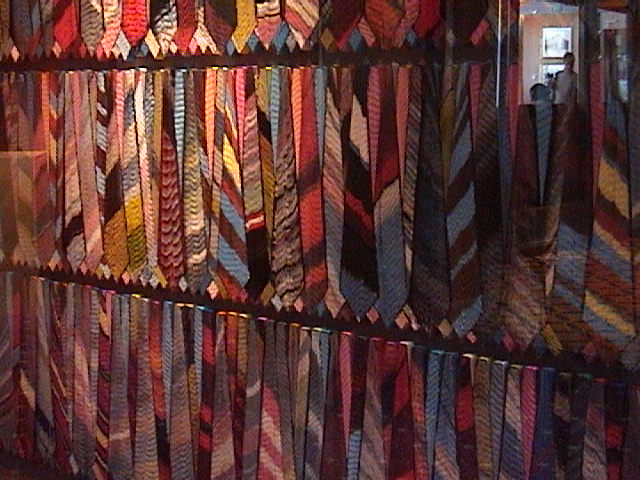The image depicts an extensive collection of neckties, arranged in a visually striking display that appears to cover a wall or panels. The ties, more than a hundred in number, are densely packed and layered over one another, creating a vibrant mosaic of patterns and colors, ranging from light and dark blues to greens, reds, pinks, oranges, yellows, and purples. They are primarily striped or patterned, each unique yet blending harmoniously in the overall arrangement. This assemblage is housed within a setting that suggests a residential space, highlighted by a small window or door opening in the top right corner through which another room is visible. The reflective surface in this area also hints at the presence of figures, possibly a person or people, adding an intriguing human element to the scene. The display’s structure includes three distinct panels – a short one at the top, a full panel with a cut-out window on the right, and a third panel at the bottom – further enhancing the layered, kaleidoscope effect of the ties against what seems to be a wooden backdrop.